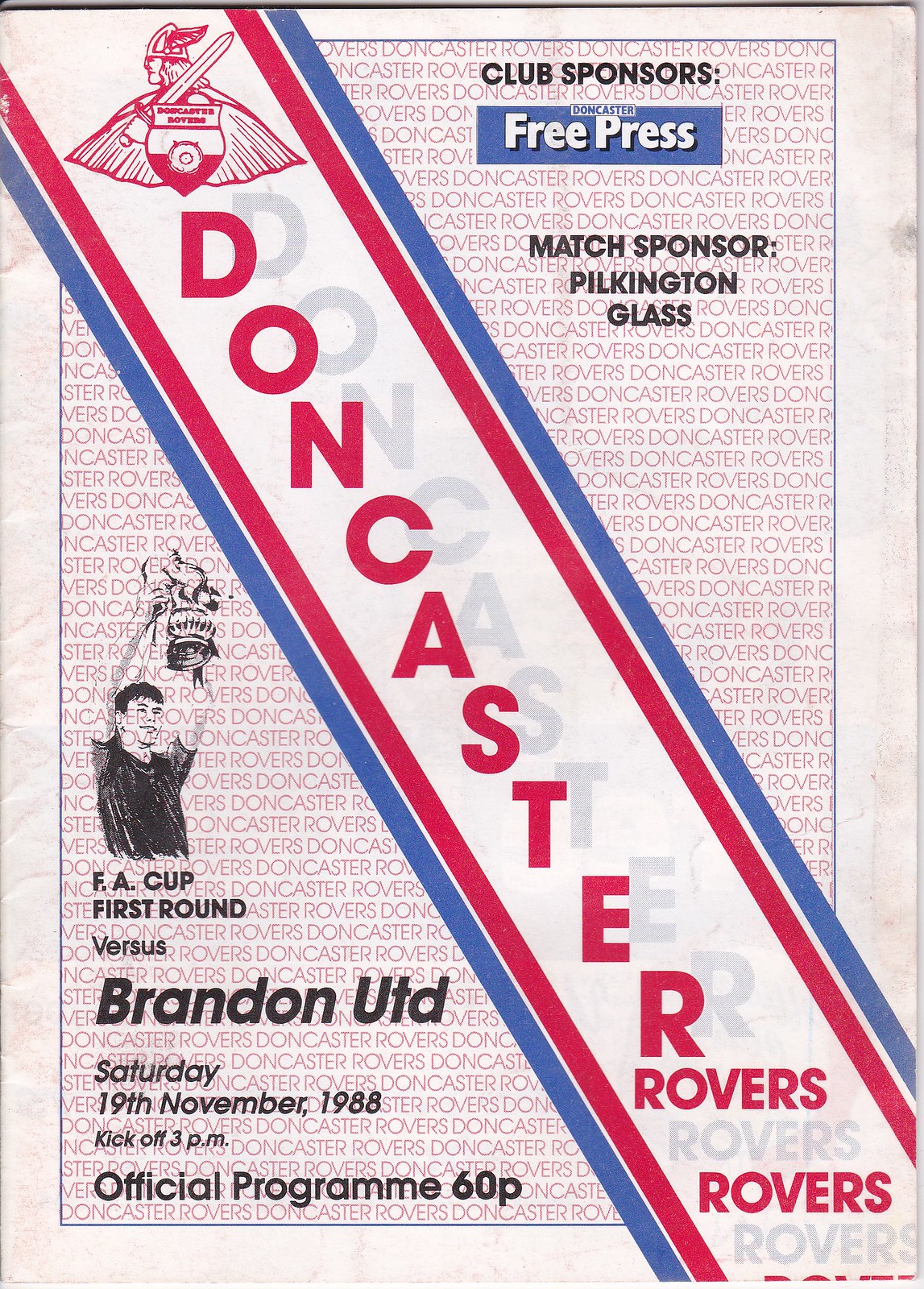The image depicts the vertically aligned rectangular cover of a light-colored program booklet for a soccer game. The background features a faded, repeating pattern of the words "Doncaster Rovers" from top to bottom. A diagonal stripe, running from the upper left to the lower right, prominently displays the name "Doncaster Rovers" in red letters, flanked by blue and red stripes. At the top of the cover, the Club Sponsor "Free Press" and Match Sponsor "Pilkington Glass" are mentioned. The team's logo, which resembles a prince in a hat with a sword in a side view, is situated above the banner. Below the diagonal stripe, there is an outline of a man holding up a trophy with bold black text stating "FA Cup First Round vs. Brandon UTD, Saturday, 19th November 1988, Kickoff 3 p.m., Official Program 60p." The spine on the left side of the program shows visible wrinkles. The cover design is simple and intended for fans attending the soccer match.